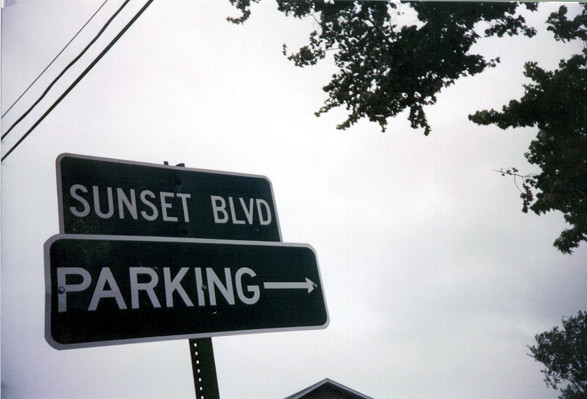A photograph captures an upward-angled view of street signs against a moody, overcast sky. The top sign prominently displays "Sunset Boulevard," while below it, a secondary sign reads "Parking" with an arrow pointing to the right. Three electrical lines stretch horizontally across the sky above and beyond the signs, contributing to the composition's linear aesthetic. On the right-hand side, tree leaves and branches subtly frame the scene, adding texture and depth. In the bottom corner of the image, the edge of a roof is just visible. The overall atmosphere is subdued, almost monochromatic due to the low lighting and muted colors, giving the impression of a black-and-white photograph. Only a small portion of the pole supporting the road signs is visible, hinting at its presence without dominating the frame.